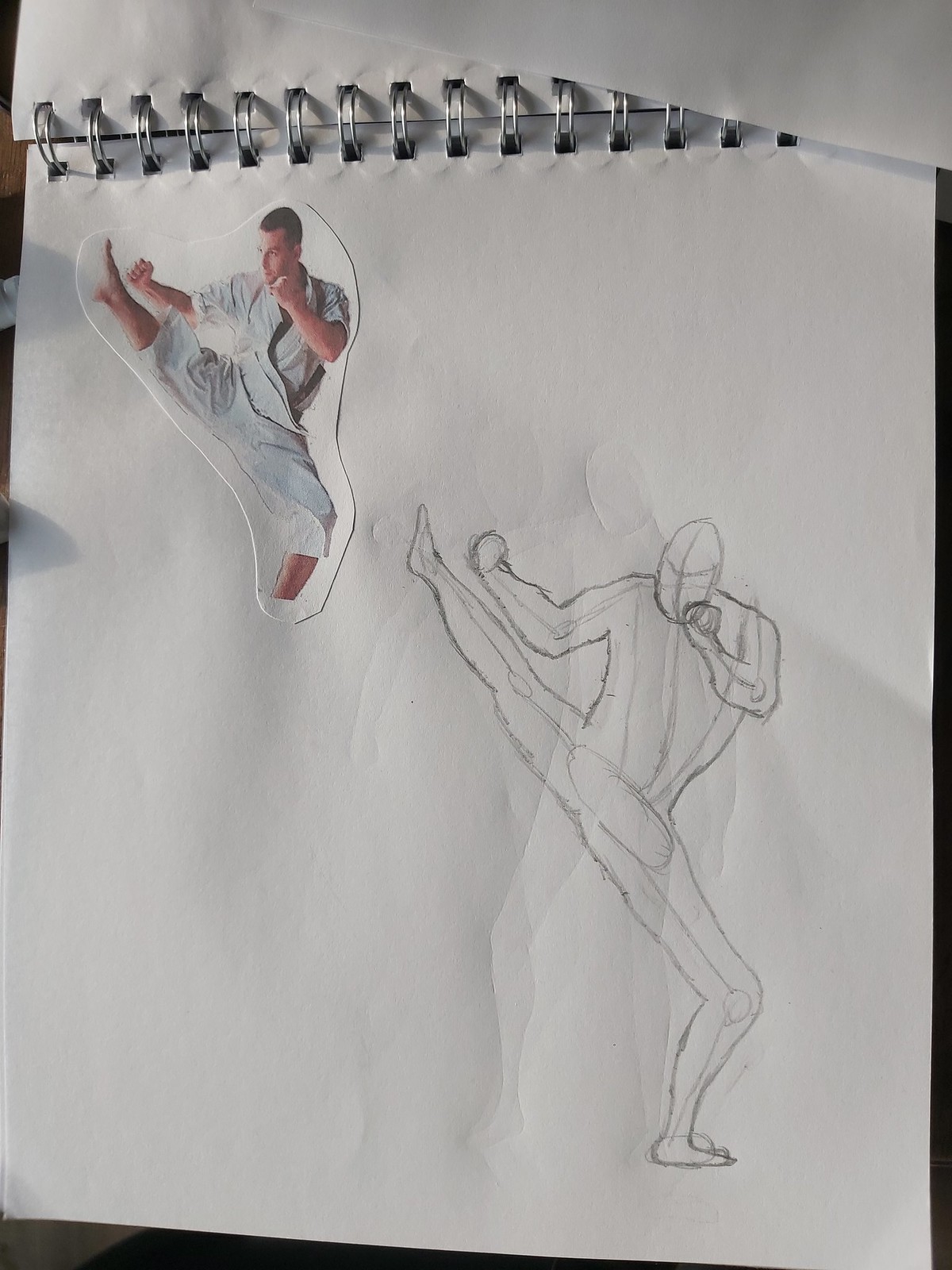In this image, we observe a close-up of a white notepad that occupies nearly the entire background. The notepad is bordered by a thin black trim visible along the right-hand side, bottom edge, and a small portion of the upper left corner. Metal rings bind the top of the notepad, indicating it is a spiral-bound notebook. 

On the top left corner of the notepad, there is a cutout image of a man performing a high kick. He is dressed in a white robe and has short black hair. His left foot is elevated in a dynamic fighting stance. Below and to the right of this cutout, there is a light gray sketch that replicates the man's pose, mirroring his body position and details with a simple outline. The entire scene is depicted on a white, square piece of paper, emphasizing the sketched and photographic elements against a clean background.